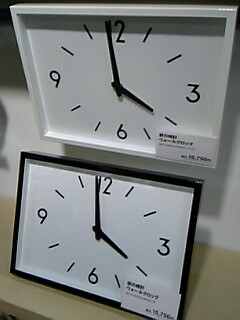This color photograph, though small, provides a detailed view of two identical rectangular clocks with distinct frames. One clock, with a black frame, is positioned on a wooden shelf, while the other, featuring a white frame, is mounted on the white wall above. Both clocks, designed to be versatile for either desk placement or wall mounting, display the same time—2 minutes before 4 o'clock. The clocks share a minimalist design with only the numbers 12, 3, 6, and 9 marked, while the remaining hours are indicated by short black lines. The identical clocks also feature small white cards affixed to the lower right corners of their faces, likely containing pricing information in non-U.S. currency and possibly written in an Asian script. Subtle shadows cast beneath each clock add depth to the image, which seems to be taken in a store setting, as suggested by the display arrangement and the visible price tags.